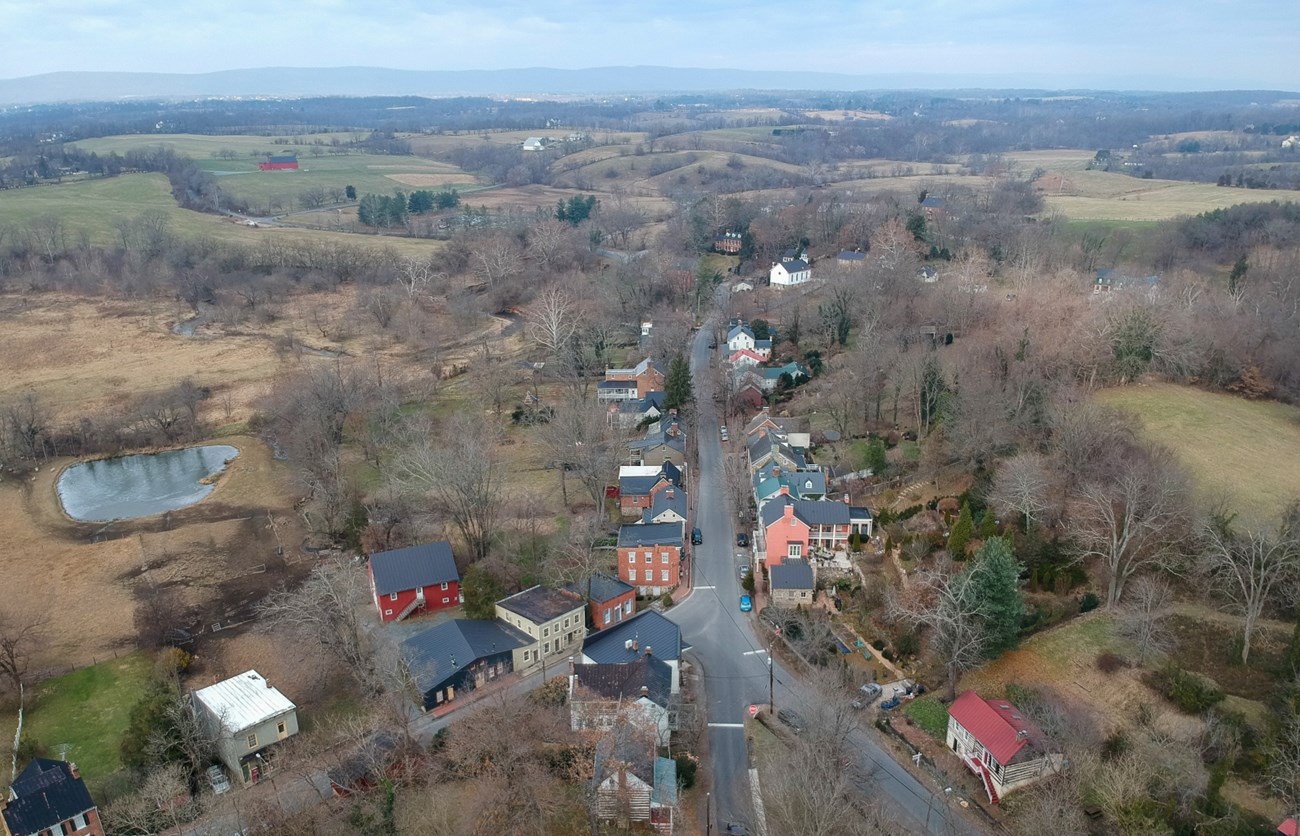This aerial photograph captures a small town nestled in a landscape that appears to be in late fall or early winter, as evidenced by the many leafless deciduous trees interspersed with evergreen trees. The town is a mosaic of red, white, orange, green, beige, and black houses, some of which may be commercial buildings. A notable feature is a winding road that starts at the bottom center and forks into three distinct paths, each lined with variously colored and roofed buildings. To the left of the image, a large pond, possibly partially frozen, emphasizes the chilly season. The backdrop includes rolling hills, open plots of land, and a distant forest beneath a light blue sky. At the very back, a red barn with a dark roof can be spotted, adding a quaint touch to the scene. The overall landscape has a brownish hue, enhancing the dreary yet serene atmosphere of the town.